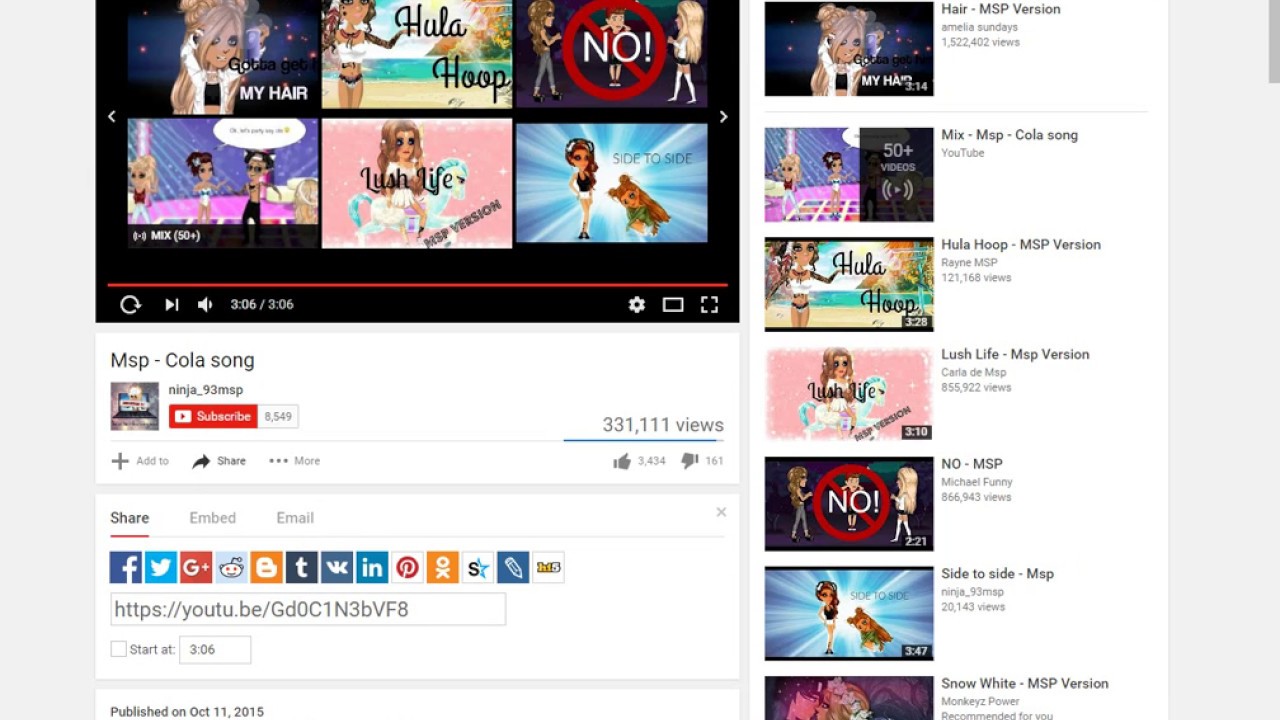This is a detailed screenshot from YouTube showcasing several video thumbnails. The first thumbnail on the left features a cartoon character with long, blonde hair, accompanied by the text "My Hair." To the right of this, there is another thumbnail titled "Hula Hoop," depicting a slender character on a beach. The subsequent thumbnail displays three people standing on a street: two women flanking a man in the center. This thumbnail features a red bullseye with the word "no" in its center, and beneath it, the text reads "MSP Cola Song." This video has garnered 331,111 views, 161 dislikes, and 3,434 likes.